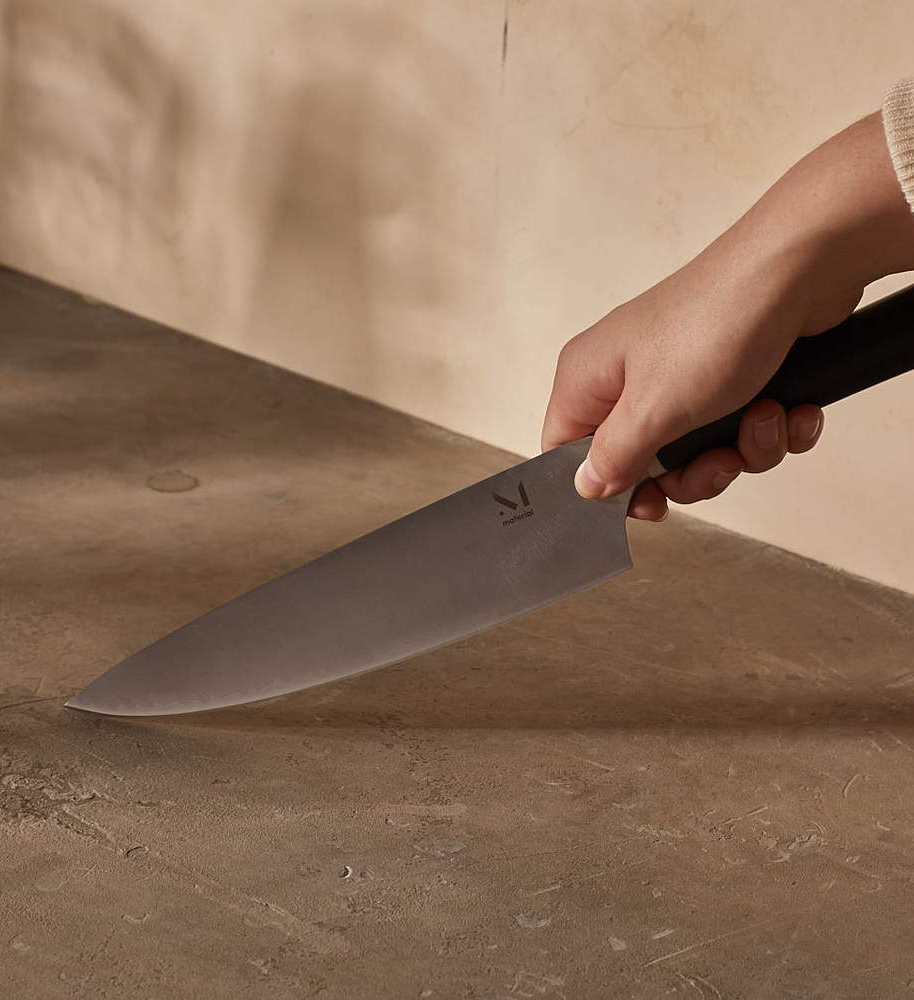The image captures a detailed scene of a person’s hand, emerging from the top-right corner, holding a large kitchen knife. The hand, likely belonging to a woman, is of a dark or light brown complexion and is clad in a tan, long-sleeved sweater. The knife, with a black, round-shaped handle, transitions into a silver blade about 8 inches long. A distinctive capital letter "M" and the word "material" are engraved near the handle. The person's thumb and forefinger are positioned on the blade, while the remaining fingers grip the handle. The knife's point rests on a textured concrete surface, marked with scratches and nicks. In the background, a light brown plaster wall completes the indoor setting, captured in a rectangular frame approximately 5 to 6 inches high and 4 to 5 inches wide. The overall scene is illuminated by daylight, highlighting the contrast between the handle's dark hue and the concrete's rough texture.